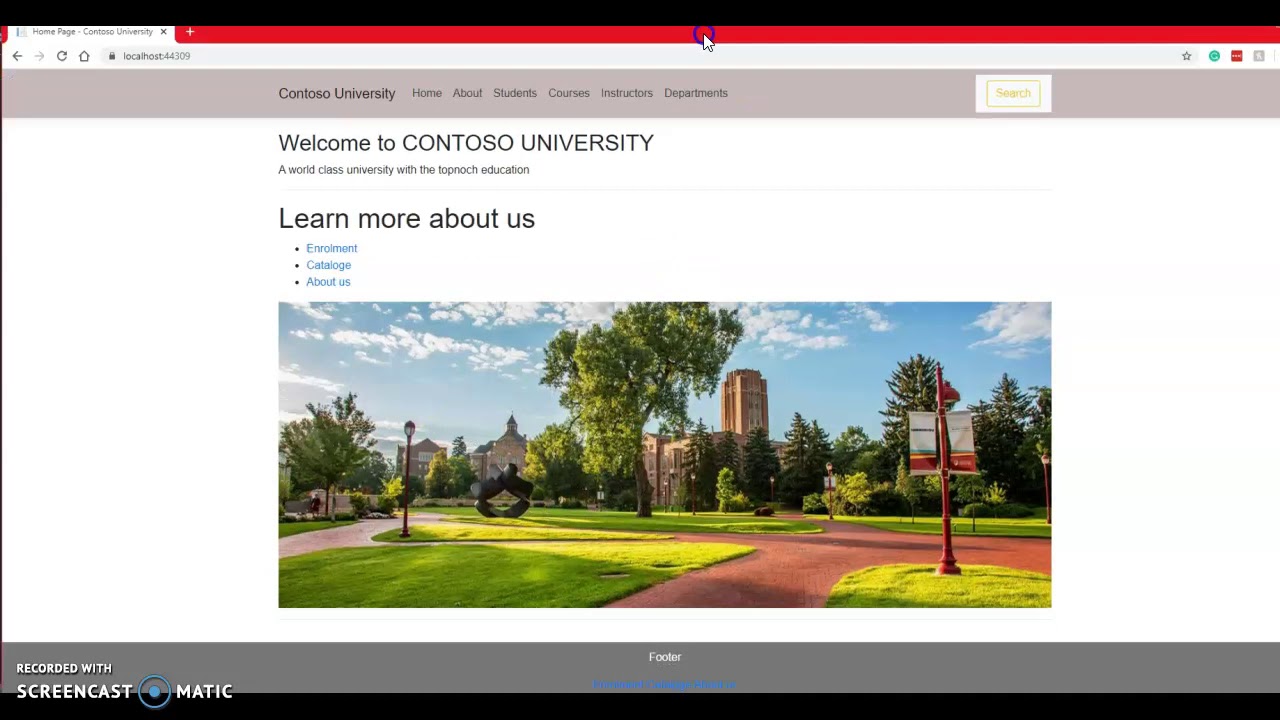The image depicts a horizontally rectangular screenshot of the Contoso University website. The primary background color is white, but narrow black horizontal banners are visible at both the top and bottom of the frame. In the upper left corner, there is a white tab, and extending from it horizontally across the top portion of the frame is a red background. Directly beneath this, the web address line is visible.

Centrally positioned, on a light gray banner, the text "Contoso University" is prominently displayed. Adjacent to this text on the same light gray banner is a navigation bar, featuring options labeled Home, About, Students, Courses, Instructions, and Departments. On the far right of this banner resides a search button.

Below the navigation bar, set against a white background, the text reads, "Welcome to Contoso University, a world-class university with top-notch education." Directly beneath this introductory text, the phrase "Learn More About Us" is written in bold, and under it, three vertical links in blue offer further navigation options: Environment, Catalog, and About Us.

The lower section of the screenshot features a large horizontally rectangular image, displaying an outdoor scene from the university campus.